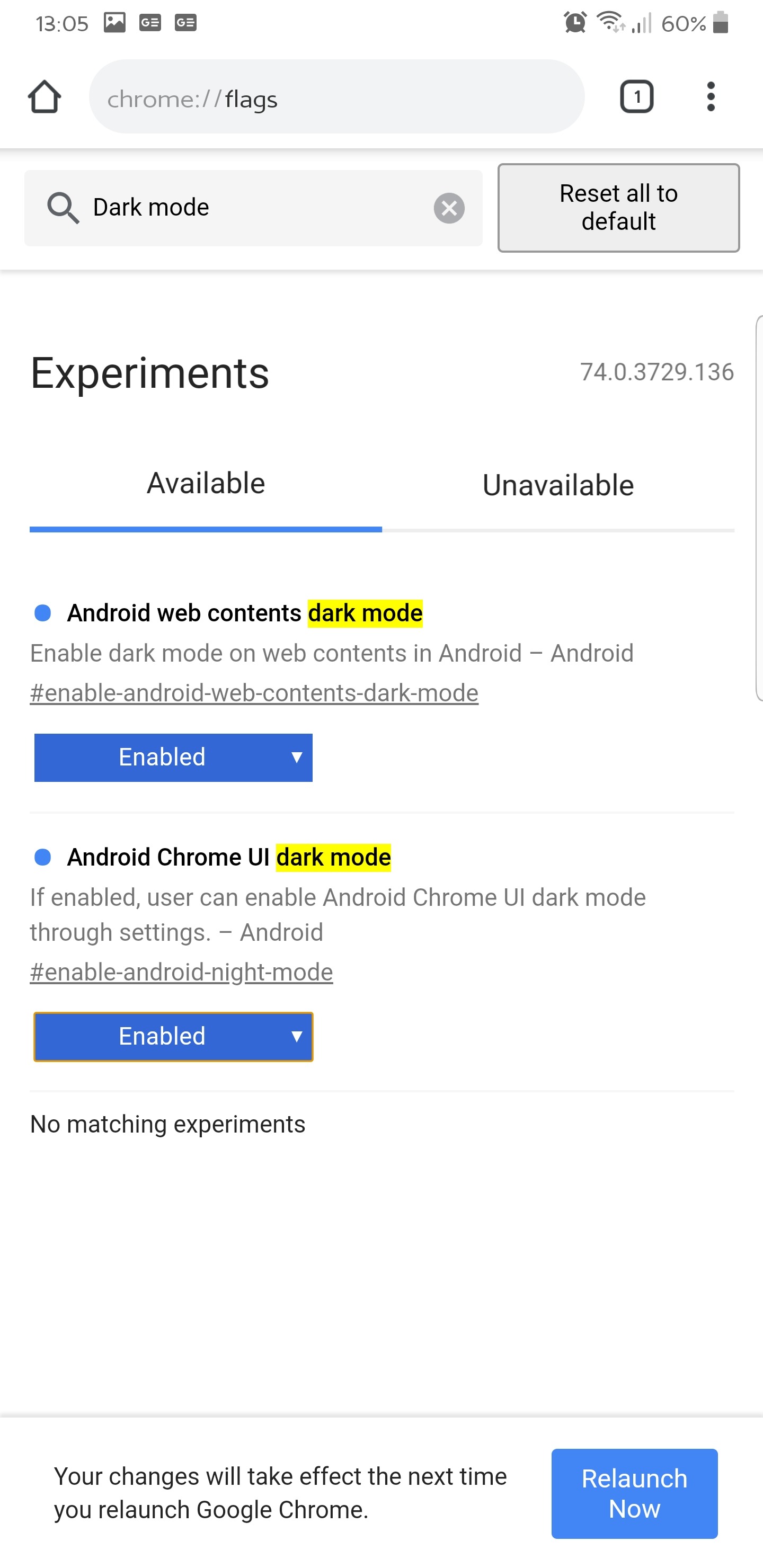In the image, a smartphone screen displays a settings page within the Google Chrome browser, particularly the "chrome://flags" section. The time shown at the top-left corner of the screen is 13:05, while the battery icon on the top-right indicates that the phone is at 60% charge. Below this, an alarm is set.

The webpage features an address bar at the top, with the URL "chrome://flags" entered. Directly beneath this, a search bar has the term "dark mode" typed in, and a "Reset all to default" button is situated to its right.

The primary focus of the screen is on the "Experiments" section, specifically experiment number 7403729136. Two tabs are shown: "Available" and "Unavailable", with "Available" being selected. Under these tabs, two specific experiments are listed:

1. "Android web contents dark mode" – This option enables dark mode for web contents on Android devices and is switched on.
2. "Android Chrome UI dark mode" – This setting allows users to enable dark mode for the Chrome user interface through the settings menu and is also toggled on.

At the bottom of the screen, there is a note stating, "Your changes will take effect the next time you relaunch Google Chrome," accompanied by a "Relaunch Now" button situated in the bottom-right corner.